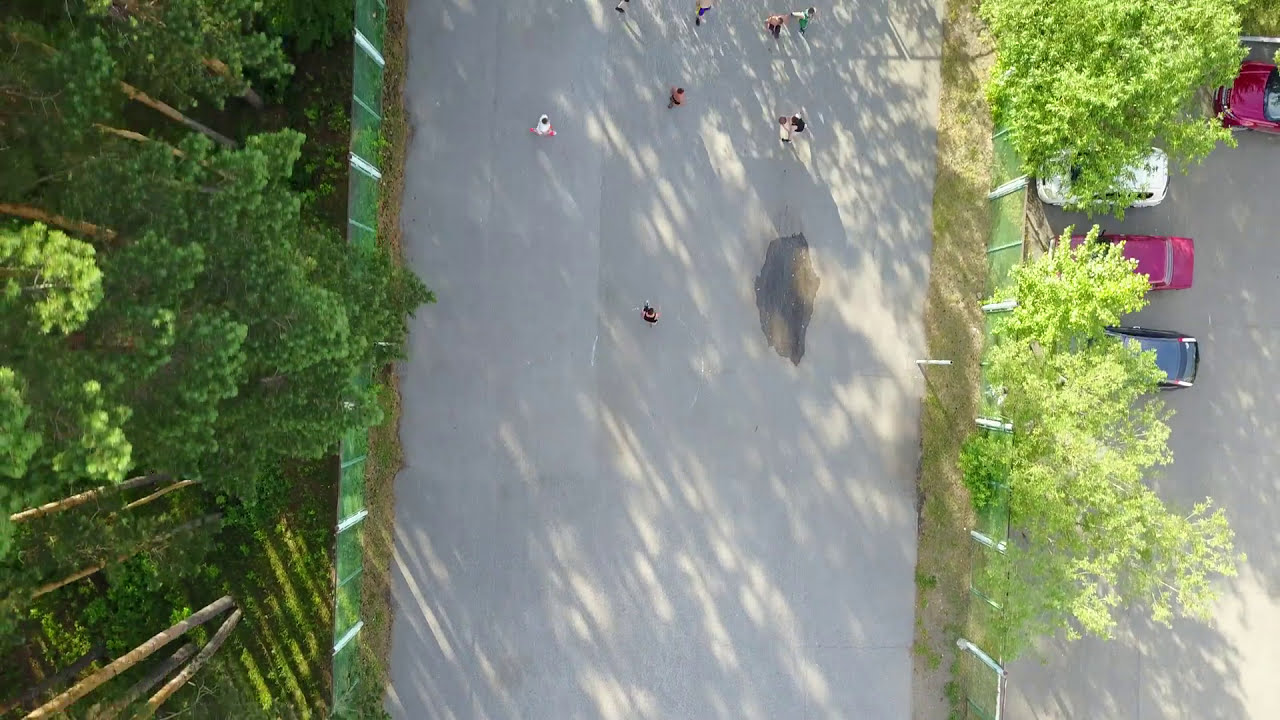This image, captured from a drone, presents a detailed bird's-eye view of a wide asphalt pathway, tannish-gray in color, stretching from the bottom to the top of the frame. The pathway is bustling with people walking in both directions. It is bordered by a greenish fence with white support beams on both sides. On the left side, the path is flanked by a dense wooded area with tall green trees and brown trunks. To the right, a smaller line of trees separates the path from an adjacent parking lot. The parking lot features cars in various colors: two red, one blue, one black, and one white. A prominent water stain can be observed in the middle of the pathway. The image, free of any text, vividly displays colors such as brown, green, black, beige, white, pink, red, and purple, contributing to the lively and detailed scene.